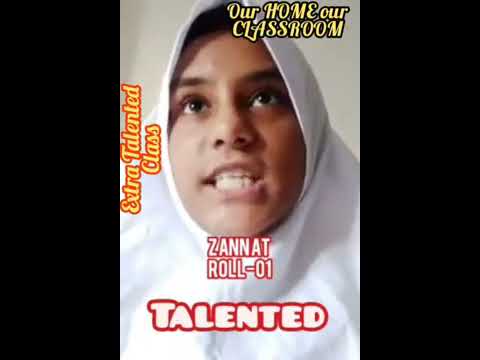The image features a young woman with an olive complexion, adorned in a white hijab. Her dark eyes are directed upwards, and she displays a wide, toothy grin with her mouth slightly open, revealing her white teeth. The screen is bordered with text: "Our Home, Our Classroom" is written prominently at the top, "Extra Talented Class" is inscribed along the left side, and at the bottom, her username "Zanatrol01" is displayed, followed by the word "talented" in balloon letters. The background of the image is entirely white, and the woman occupies most of the frame, visible from the shoulders up, though her shoulders are covered. The overall style suggests it might be a video screenshot taken in a home setting.